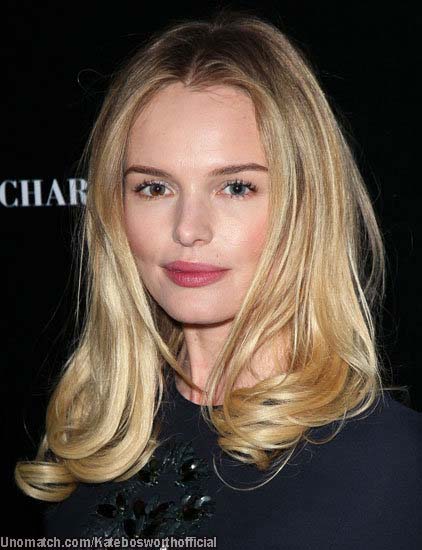The image features a woman in her 30s with long blonde hair that has loose curls at the ends. She has blue eyes, darker eyebrows, and is wearing pink lipstick. The woman is dressed in a dark blouse, decorated with sparkling black floral elements under the collar. She gazes directly into the camera with a neutral smile on her face. The backdrop is a solid black background with the letters "C-H-A-R" in white, positioned at eye level to her left. The bottom of the image displays the text "UnoMatch.com Kate Bosworth Official."